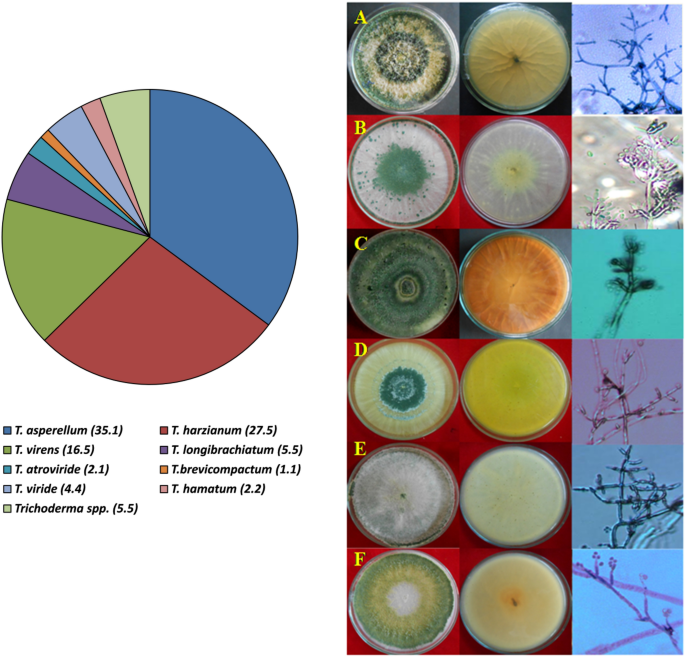The image showcases a detailed scientific analysis involving petri dishes and bacterial growths. Twelve petri dishes (labeled A to F with corresponding numeric identifiers) exhibit vibrant and varied bacterial colonies; one is bright yellow, another orange, a third green and white, while others display combinations of white and purple or shades of green and yellow. Each petri dish is paired with close-up microscopic views of the bacterial formations, progressively zooming in to reveal intricate cellular structures. To the left of these dishes, a pie chart, segmented and color-coded in maroon, green, blue, pink, purple, and orange, provides data on the bacterial strains shown in the petri dishes, with each color representing a different type of bacterium. Beneath the pie chart, a key explains the significance of each color, correlating the bacterial types to their respective percentages. The vibrant colors and detailed close-ups highlight the diversity and complexity of the bacterial samples under examination.